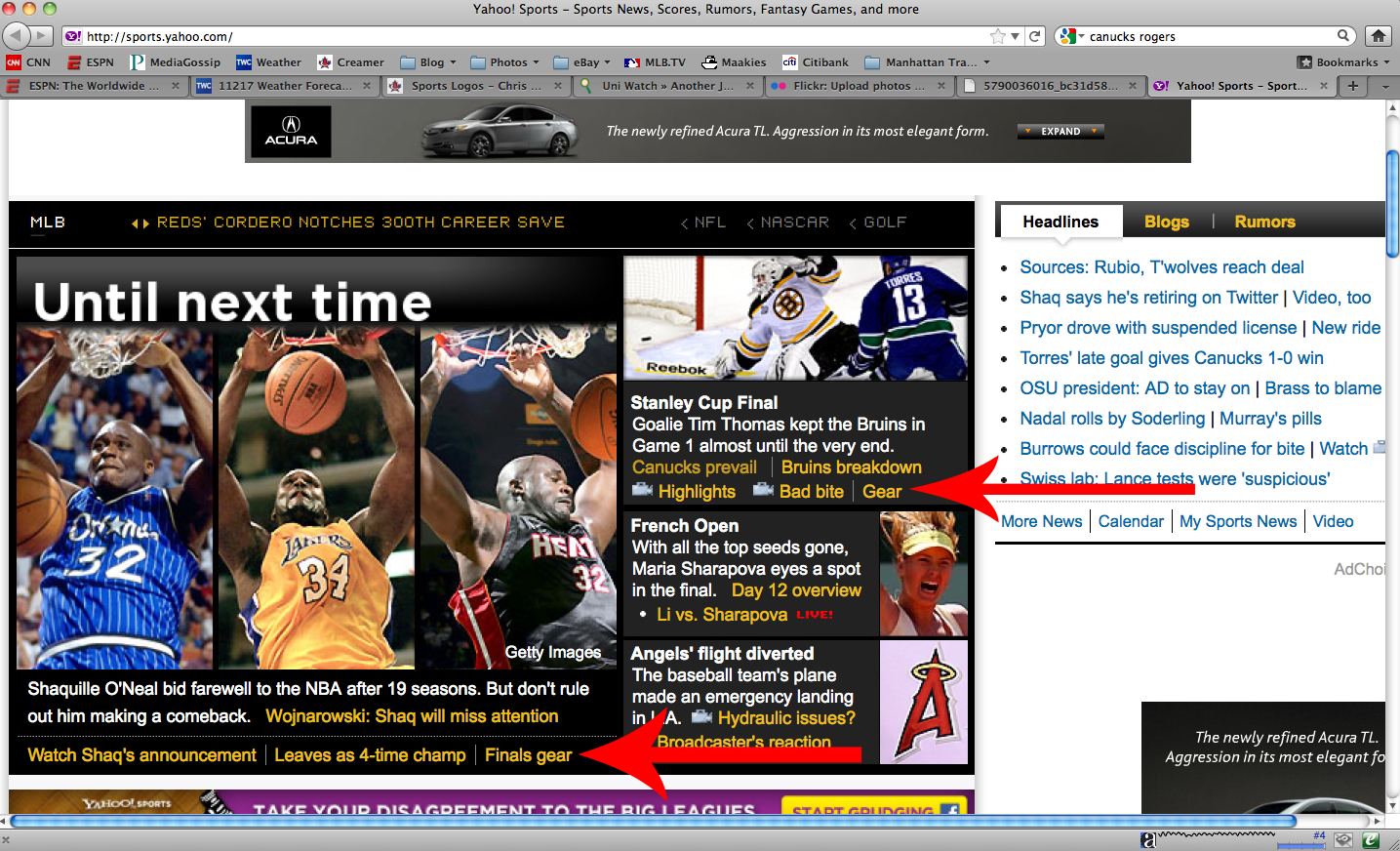This image captures a full screenshot of a sports-themed website, viewed on what seems to be an Apple-based computer. In the top left-hand corner, distinctive red, orange, and green dots indicative of Mac OS can be seen, confirming the operating system. The website is identified as Yahoo Sports, prominently displaying its logo and tagline: "Sports News, Scores, Rumors, Fantasy Games, and more."

Just below the header, a user interface element includes two navigation arrows: a green arrow highlighted to the left and another arrow in a square box pointed to the right, flanking a central search bar that utilizes Yahoo for searches. To the right of this primary search bar, there is an additional search bar labeled with the Google logo, alongside a house icon which likely serves as a home button.

Towards the upper part of the screen, a carousel of bookmarks lists popular websites such as CNN, ESPN, among others. The central focus of the screen is a dynamic display featuring basketball legend Shaquille O'Neal in various dunking actions, showcasing his time with the Orlando Magic, Los Angeles Lakers, and Miami Heat.

Additionally, the interface includes two prominent red arrows: one large arrow pointing to the left, directing attention towards 'gear,' and another large red arrow also pointing to the left, highlighting 'finals gear.' On the right side of the screen, there is a section dedicated to headlines, featuring bullet-pointed information, with tabs for blogs and rumors adjacent to it, providing comprehensive sports news and updates.